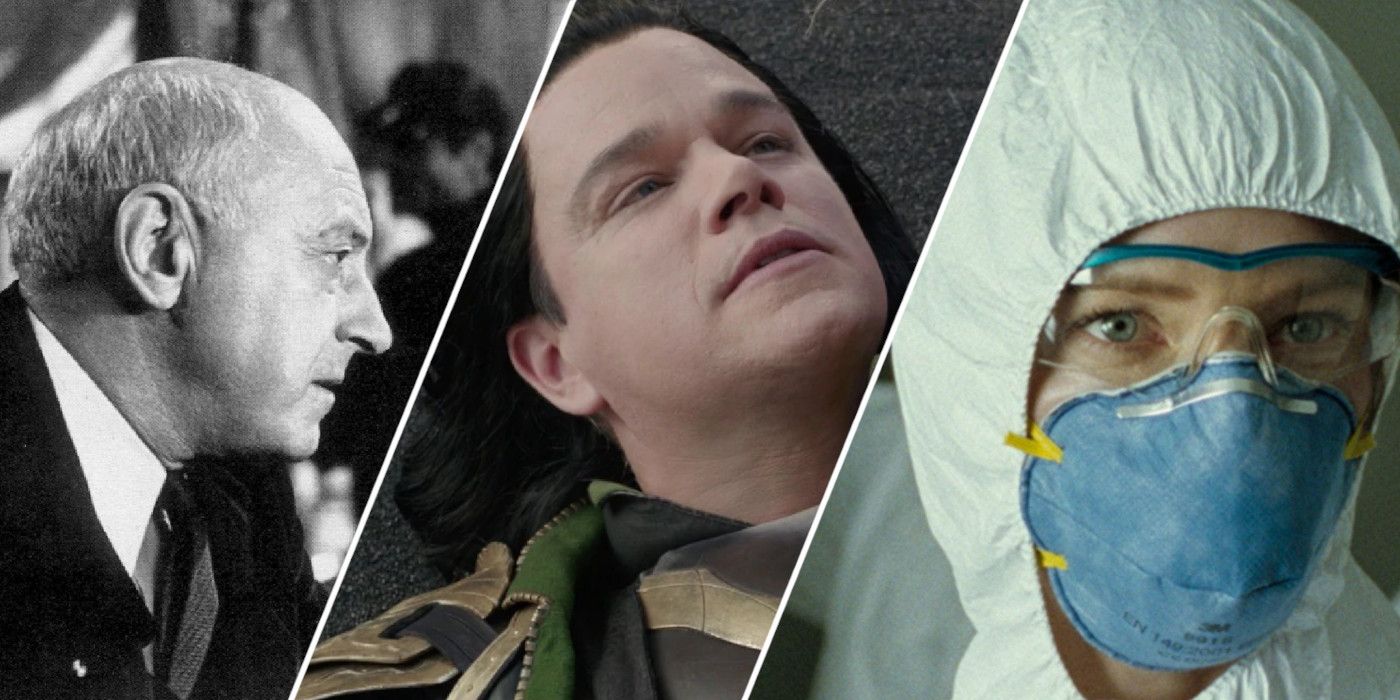The image features a collage of three distinct photographs, divided by a diagonal white line swooping downward from right to left. In the center, there is a color photograph of Matt Damon dressed as Loki from the Marvel films; he appears to be lying on the floor, looking upward with a pensive expression, his long black hair spread out beneath him. To the right, a close-up shot captures Cate Blanchett, possibly in a scene from Hannibal. She is wearing a protective blue surgical mask, clear safety goggles, and a white full-body coverall, resembling attire one might wear in a medical setting to avoid contamination. On the far left, a black-and-white image depicts an unidentified male figure in profile, dressed in a white button-down shirt and a suit jacket. The man, who has a thin hairline with most of his remaining hair in a horseshoe pattern around his head, directs his gaze towards the right, his large ears and pointy nose prominently visible.